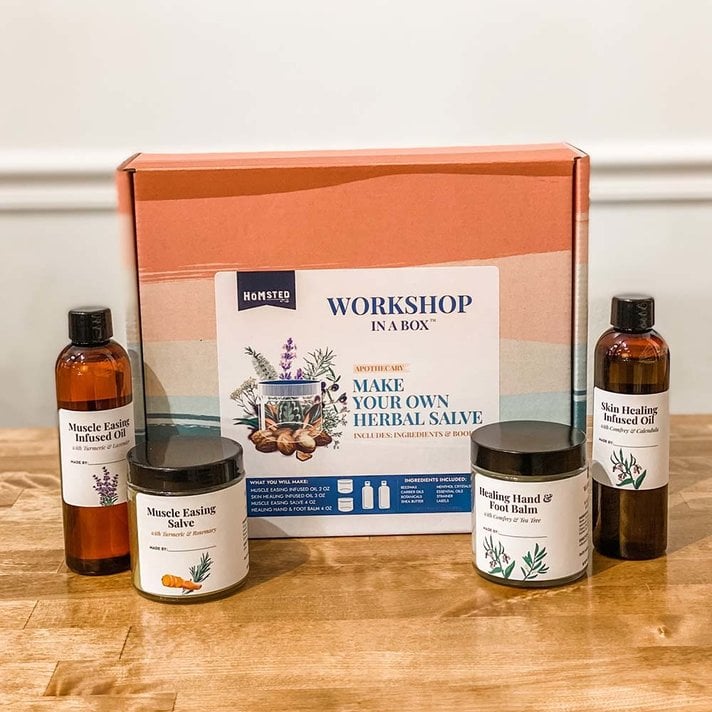In the photograph, a collection of herbal salves and oils is displayed on a medium-finished wooden table against a plain white wall. At the center, there is a box labeled "Homestead: A Workshop in a Box," adorned with neutral orange and green stripes, featuring a white label in the middle. The label highlights the kit's purpose with the text "Make Your Own Herbal Salve," and an image of a small container surrounded by herbs.

Flanking the box are four dark brown opaque bottles. Each bottle is distinctly labeled: one reads "Muscle-Easing Infused Oil," another "Muscle-Easing Salve," the third "Healing Hand and Foot Balm," and the fourth "Skin-Healing Infused Oil." These items suggest a comprehensive kit for creating and using various herbal topical treatments. The overall aesthetic of the image is characterized by neutral tones, reinforcing the natural and handcrafted theme of the products.